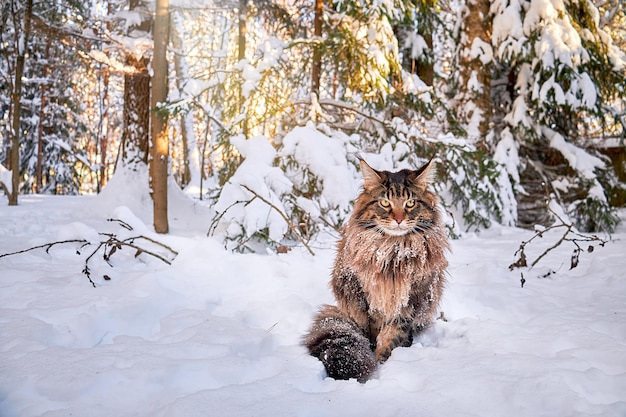A fluffy, long-haired cat with an orange-brown coat and black markings sits calmly in a deep, snowy landscape. Its yellow eyes, white whiskers, and white-tipped mouth stand out against the snowflakes dusting its fur. The cat's ears are perked up, and it looks attentively to its upper left, while its bushy, mostly black tail curls around to the front. Surrounding the cat, snow blankets the ground and nearby broken tree branches. In the background, a dense forest of evergreen trees is heavily laden with snow, their branches gleaming with a yellowish hue from the sunlight. The peaceful scene showcases the cat's resilience amidst a tranquil, wintry wonderland.